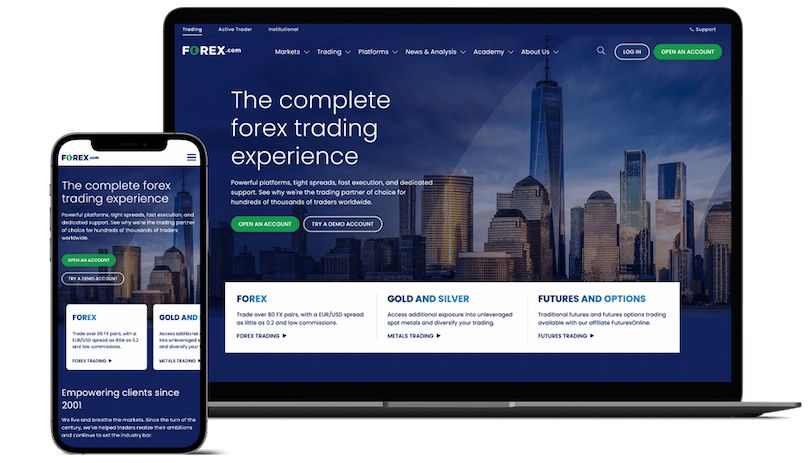This advertisement showcases the trading platform 4x.com, presented on a laptop and a cell phone. The image features a clean, white background, emphasizing the devices and their screens. Positioned on the right side of the image, the open laptop, resembling a MacBook Air, displays a blue-themed background with "4x.com" prominently in the upper left-hand corner. The font is white, with the exception of the letter "O" which is highlighted in green. To the immediate left of the laptop is a cell phone, mirroring the laptop's screen layout but adapted for a mobile format. Both screens feature the text "The Complete 4x Trading Experience – Foreign Exchange Currencies."

Key interactive elements are present on both screens, including green and blue clickable ovals labeled "Open an Account" and "Try a Demo Account," respectively. Additional informational boxes direct users to learn more about trading 4x, gold and silver, and futures and options. This ad targets individual investors interested in trading various financial instruments, emphasizing accessibility and a comprehensive trading experience.